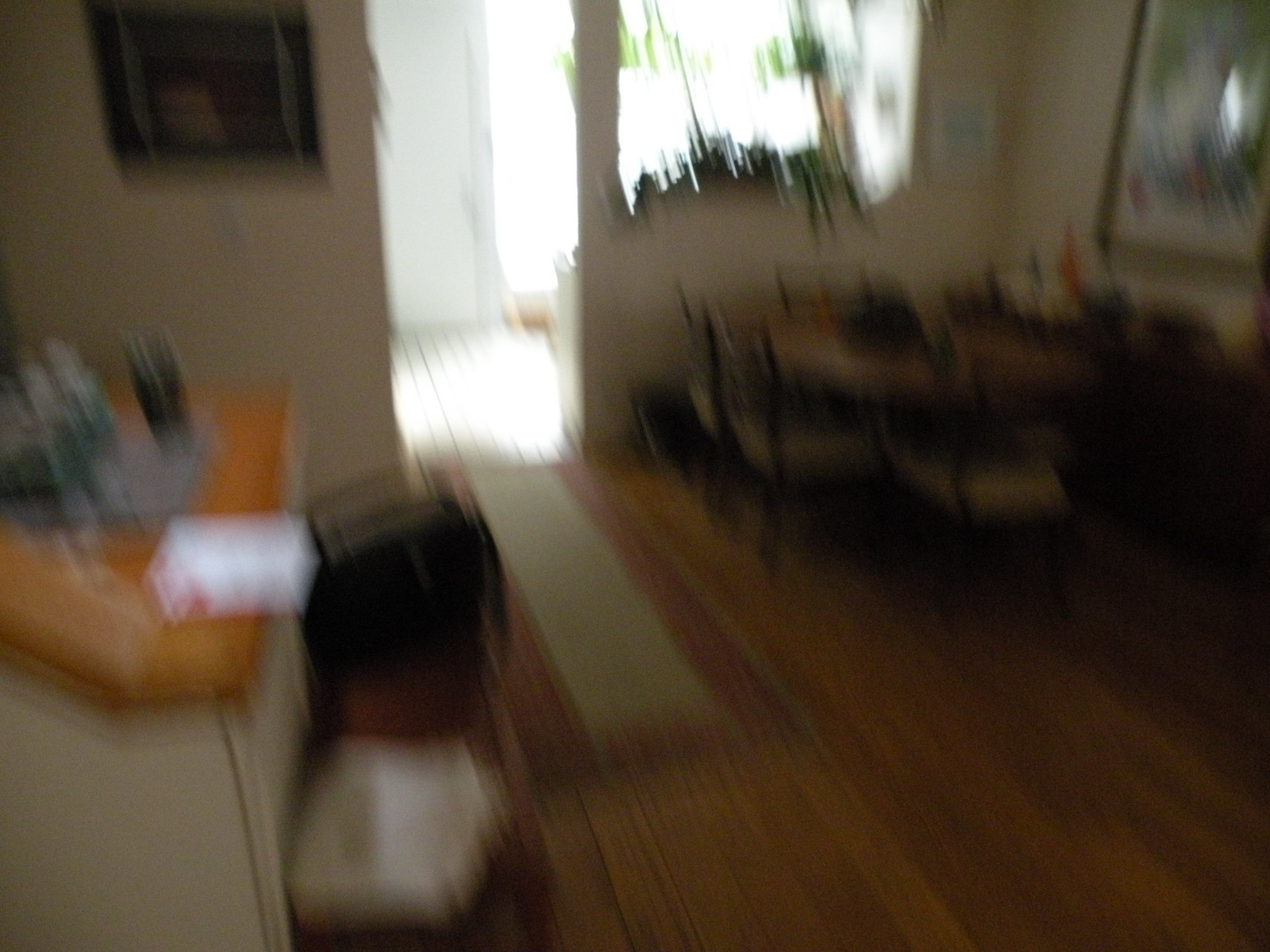Blurry and out-of-focus, the photograph reveals a scene marked by motion, suggesting that the camera was shaken during the shot. Despite the blur, several details of what appears to be a living and dining space are discernible. The image captures a wood-grain floor, an elegant dining table surrounded by chairs, and a throw rug at the entryway that leads into a small foyer with a tiled floor. 

To the left, a counter is visible, possibly serving as a prep area or kitchenette, featuring a silver rectangle that might be a hot plate. Further details include artwork adorning the left side and a bright beam of sunlight piercing through a doorway in the center. The scene is complemented by the subtle outlines of items on the floor, such as totes or shopping bags, adding to the lived-in ambiance of the space.